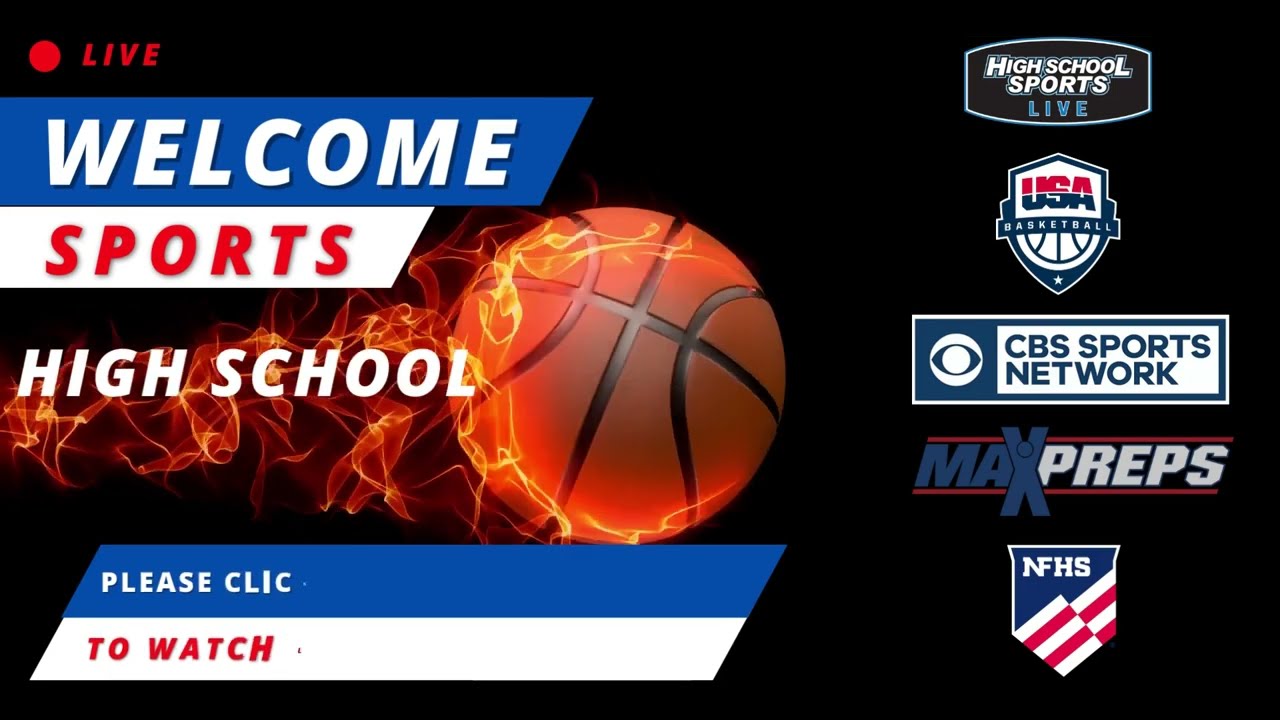The image is a dynamic advertisement for high school basketball. Set against a black background, the center features a vibrant basketball engulfed in flames, emphasizing intensity and motion. Flames shoot off to the left edge of the picture. In the upper left-hand corner, there's a red dot accompanied by the word "LIVE" in red print. Below this, a blue banner in all caps white print reads "WELCOME." Directly beneath this banner, another white banner in red capital letters states "SPORTS."

Flanking the basketball, the phrase "HIGH SCHOOL SPORTS LIVE" appears, with additional mentions of "USA BASKETBALL," "CBS SPORTS NETWORK," "MAX PREPS," and "NFHS," the latter accompanied by a logo featuring a shield and an American flag. Below the basketball, a blue banner prompts viewers with "PLEASE CLIC," followed by a white banner instructing "TO WATCH." The image is filled with various banners and emblems, bringing together elements of sports networks and organizations to highlight an exciting high school basketball event.